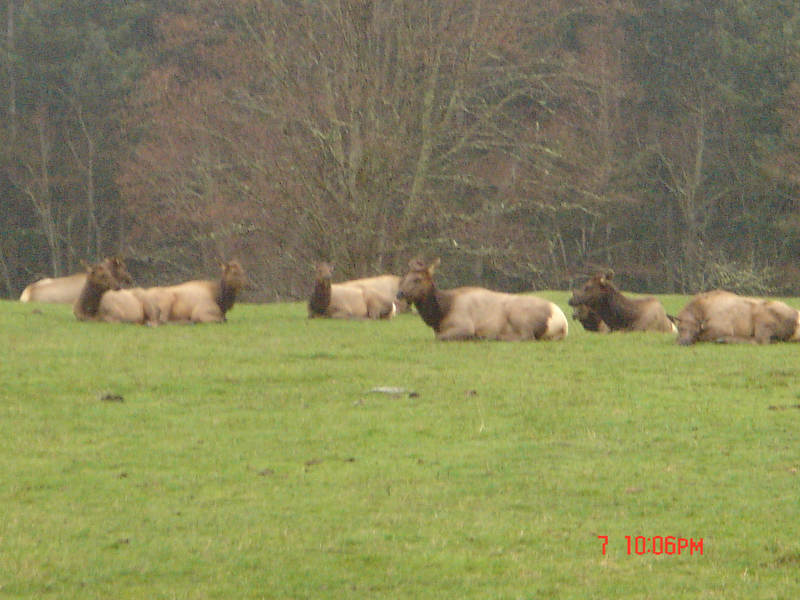In this slightly blurry outdoor photograph taken during daytime under light haze, a group of six brown animals, possibly cattle, is lying on a green grass field. These animals exhibit a light tan body with darker brown heads and pointy ears. They are mostly lying in profile with their heads oriented to the left, except for two animals on the far left facing the opposite direction. The background features a mix of tall trees with green, brown, and tan leaves, appearing sparse and giving a fall-like ambiance. The image’s slight out-of-focus and grainy nature makes it challenging to identify finer details of the animals or the precise vegetation type. A red time stamp "7 10.06 PM" overlays the lower right corner.